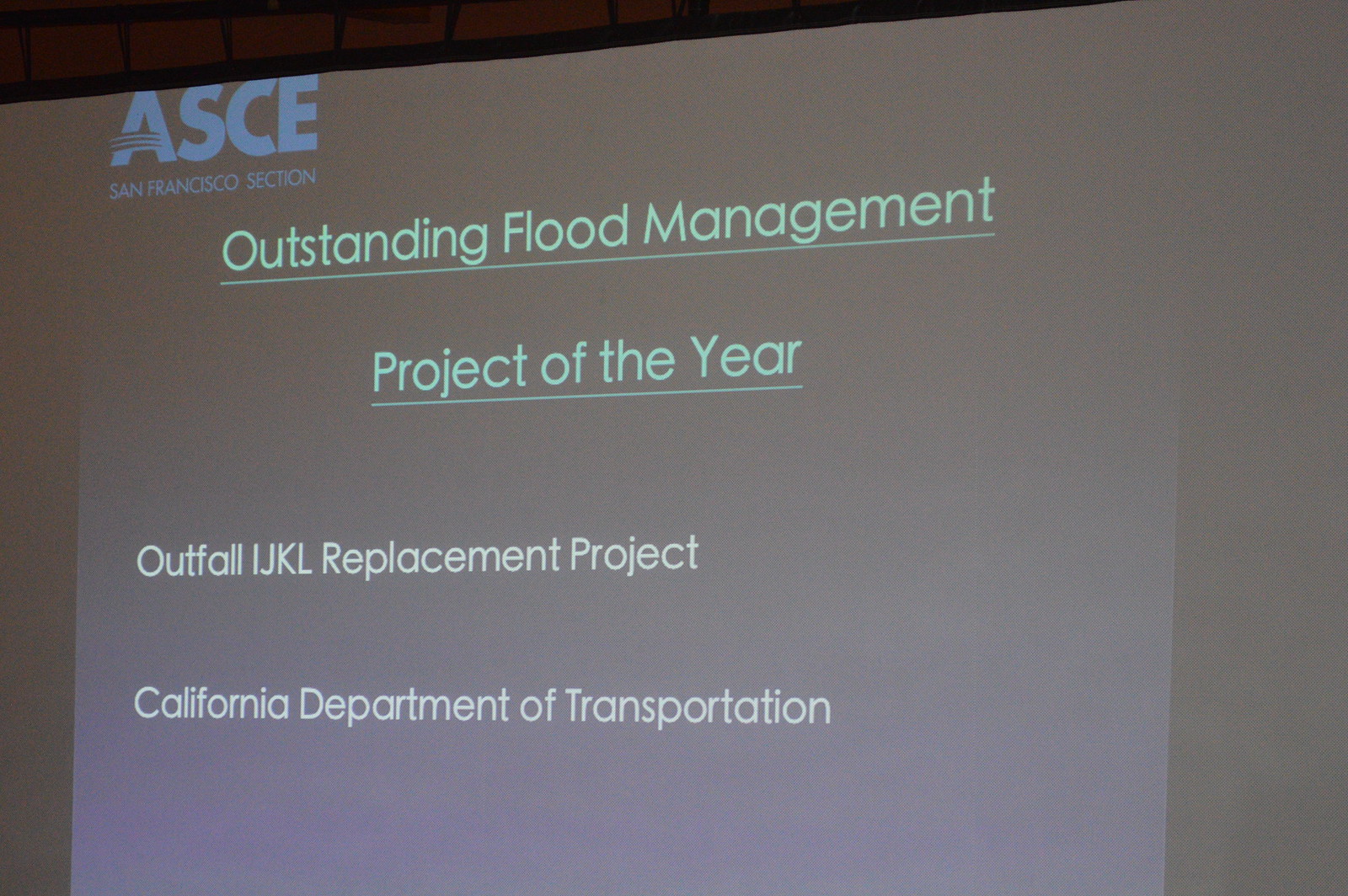This photograph captures a large projection screen at a business conference, possibly for a high-profile company like Apple or Microsoft. The central image is a PowerPoint presentation slide with a black background. In the top left corner, bold blue capital letters spell out "ASCE," with "San Francisco Section" directly underneath in smaller text. Below that, a light green title reads "Outstanding Flood Management Project of the Year," with the phrase underlined for emphasis. Further down, white text lists significant details, beginning with "Outfall IJKL Replacement Project" and followed by "California Department of Transportation." The screen's right and left sides are shadowed, making the central content more prominent and suggesting the use of an overhead projector in a conference setting.